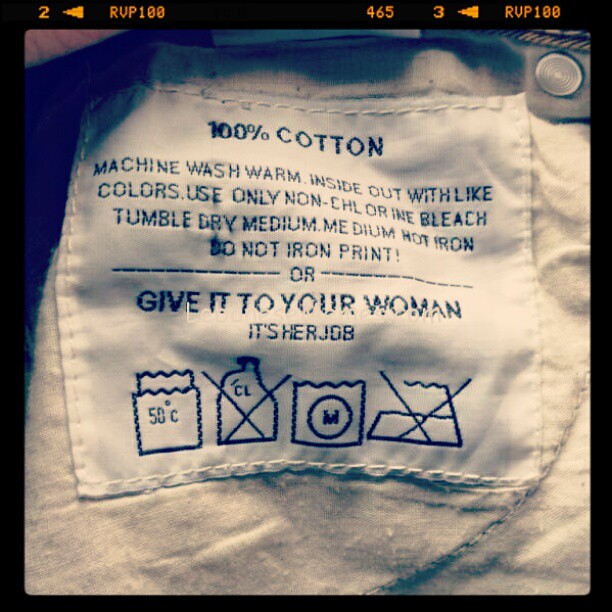The image shows a close-up of a sewn-in label inside a light-colored pair of pants, which appears to be a pocket. The label, bordered by a black trim at the top, contains detailed washing instructions embroidered in black, all-capital letters: "100% COTTON, MACHINE WASH WARM INSIDE OUT WITH LIGHT COLORS, USE ONLY NON-CHLORINE BLEACH, TUMBLE DRY MEDIUM, MEDIUM HOT IRON, DO NOT IRON PRINT OR GIVE IT TO YOUR WOMAN, IT'S HER JOB." The instructions are complemented by various care symbols, including a 50 degrees Celsius indicator, a crossed-out chlorine bleach symbol, and a crossed-out iron symbol. Visible in the top right corner of the image is a button, possibly part of a button fly, hinting at the functional design of the pants. Significant numeric and symbolic elements, such as "465" and "RUP 100," appear in yellow at the upper left and right corners, providing additional garment details. The photographed label layout shows a blend of functional information with a controversial and outdated remark about gender roles.